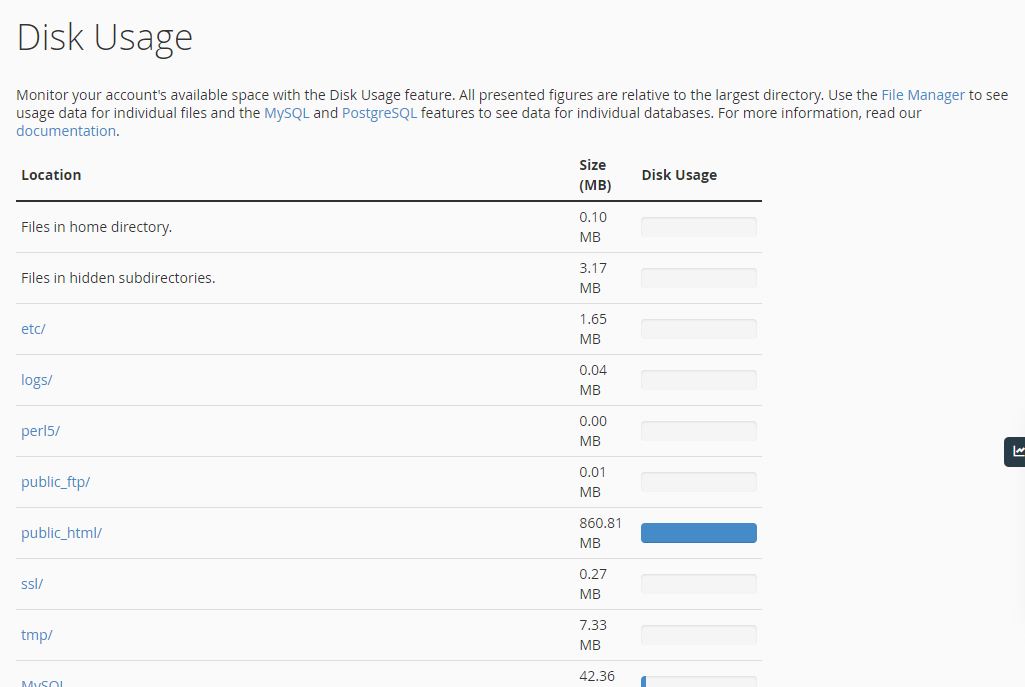The image captures a screenshot of a disk usage monitoring interface. The background is white with gray text at the top. The title "Disk Usage" is displayed on the left, followed by a brief description: "Monitor your account's available space with the disk usage feature. All presented figures are relative to the largest directory. Use the file manager to see usage data for individual files and MySQL and PostgreSQL features to see data for individual databases. For more information, read our documentation." The terms "documentation," "file manager," "MySQL," and "PostgreSQL" are highlighted in blue, indicating they are clickable links.

Beneath the description, there are column headers labeled "Location," "Size (MB)," and "Disk Usage." A list of directories follows, detailing their respective disk usage. The entries include:

- **Files in home directory**: 0.10 MB
- **Files in hidden subdirectories**: 3.7 MB
- **ETC/**: 1.6 MB (displayed in blue)
- **logs/**: 0.04 MB (displayed in blue)
- **ER15/**: 0 MB (displayed in blue)
- **public_ftp**: 0.01 MB (displayed in blue)
- **public_html**: 860.81 MB, indicated with a large blue usage bar
- **SSL/**: 0.27 MB (displayed in blue)
- **tmp/**: 7.33 MB (displayed in blue)

The list continues, but the visibility of an entry showing 42.36 MB is partially obscured.